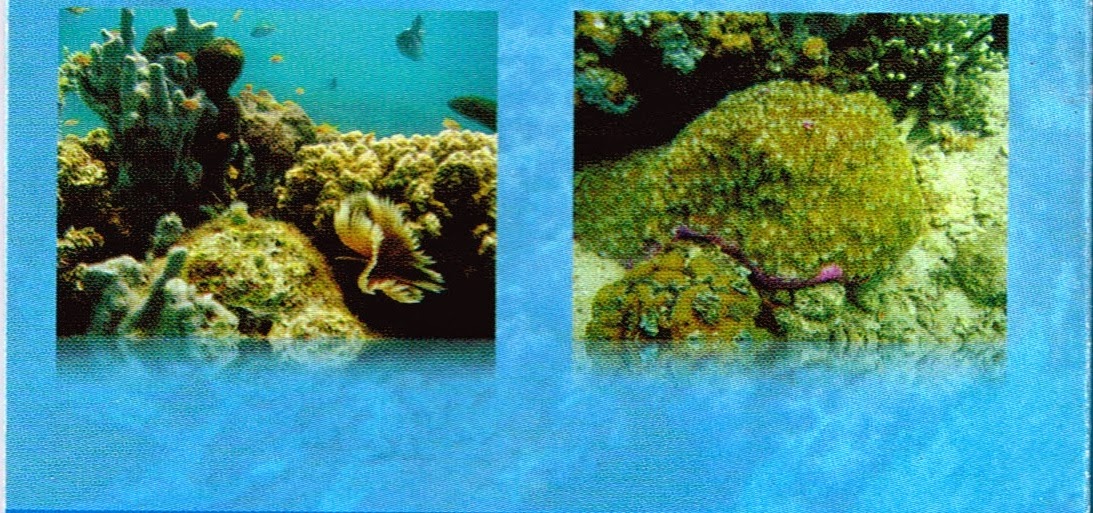The image depicts two side-by-side underwater photographs set against a light blue background. The left photograph showcases a vibrant coral reef teeming with marine life. The clear blue water allows a view of several fish swimming near the reef, with little gold fish staying close to it and a few larger fish exploring the surroundings. The reef is populated with colorful species, exhibiting hues of turquoise, tan, orange, green, and purple, and bordered by underwater greenery. The right photograph offers a view of the ocean floor, featuring sand, scattered rocks, sea moss, and underwater plants. Prominently, there are sea urchins attached to one of the rocks. The overall grainy texture of the photographs gives them a vintage feel, enhancing the sense of an underwater exploration scene.